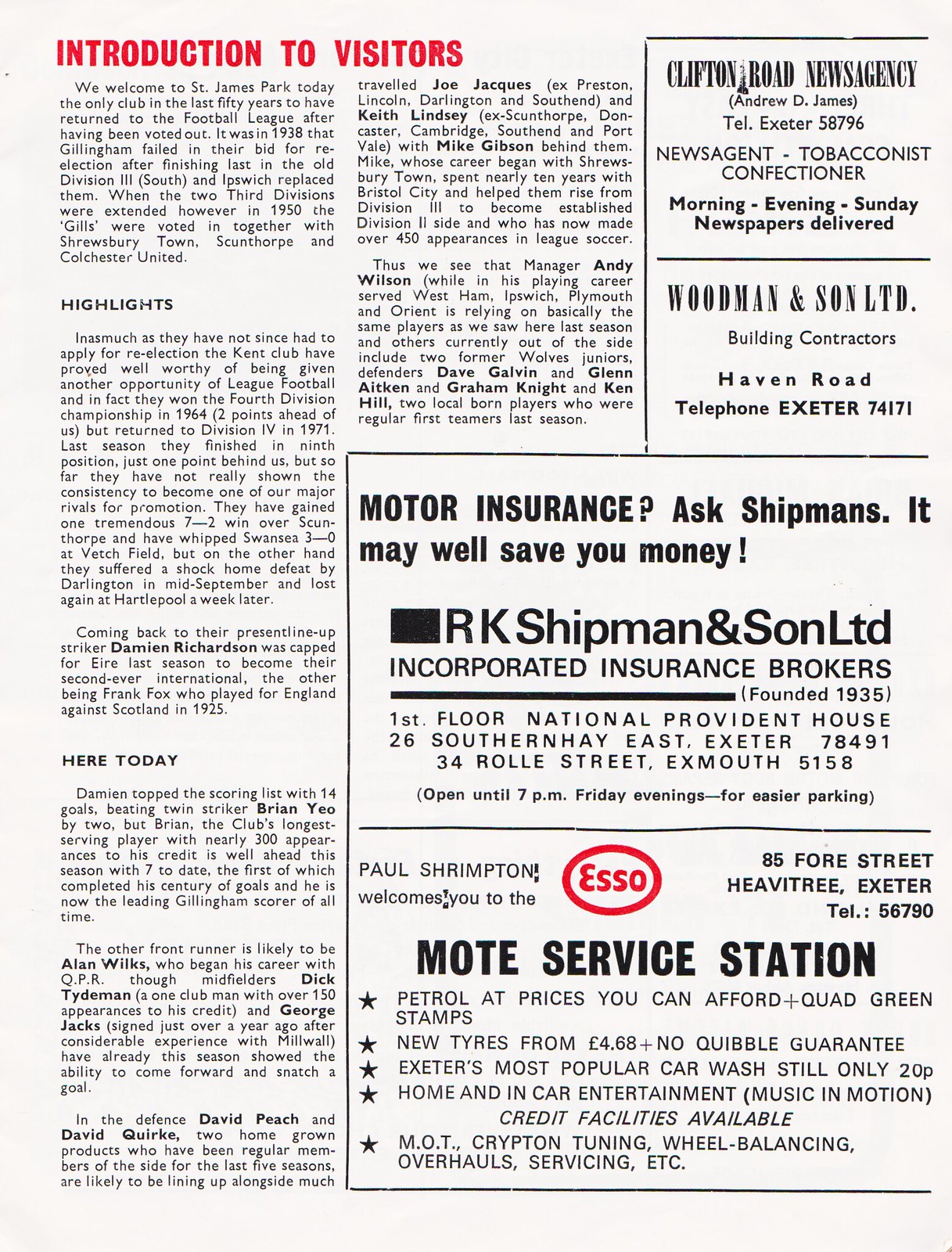The image is a tall rectangular flyer or advertisement from a magazine or newspaper, with a background that is a light off-white color resembling paper. In the very top left corner, large red font reads "Introduction to Visitors." Beneath this title are multiple columns of text in much smaller black font. The left column welcomes visitors to St. James Park, highlighting it as the only club in the last 50 years to have returned to the football league after being voted out. The text recounts the history of Gillingham, which failed in its bid for re-election in 1938 but was voted back in 1950 along with Shrewsbury Town, Scunthorpe, and Colchester United. This section also includes highlights and information under titles such as "Highlights" and "Here Today," describing today's match participants, including details about the players, managers, and junior defenders.

In the top right corner, there are two small advertisement sections bordered by black lines. The top ad, in thick all-capital letters, reads "Clifton Road News Agency," with additional information beneath it. Below this, in fancy all-capital letters, another ad reads "Woodman and Son LTD." Towards the bottom right, there are two larger advertisements; the first begins with "Motor Insurance? Ask Shipments. It may well save you money." Other sponsors listed include RK Shipman and Son Limited, Woodman and Son Limited, Clifton Road News Agency, and Mote Service Station. These sponsors are likely funding the printing of the flyer to provide information about the team's highlights and today's events.